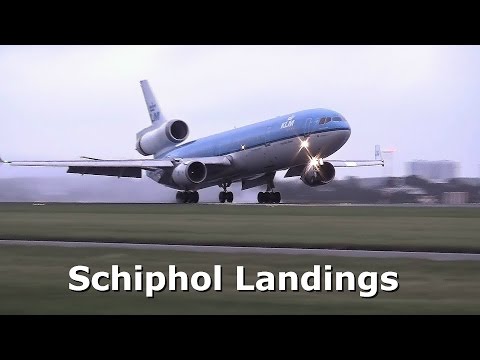The image depicts a jumbo jet, possibly a KLM aircraft, either landing or taking off on a runway. The plane's top is a dark blue, transitioning to a brownish-gray or silver on the underside, with gray engines and outstretched wings. There are bright yellow lights on the underbelly, and the wheels are down, touching the runway. The runway is bordered by green grass, and some blurry buildings appear in the background. The sky above is partly cloudy with varying shades of blue and gray, indicating an overcast day. The entire scene is framed by thin horizontal black strips at the top and bottom. White text reading "Schiphol Landings" is placed in the foreground against the grassy area.